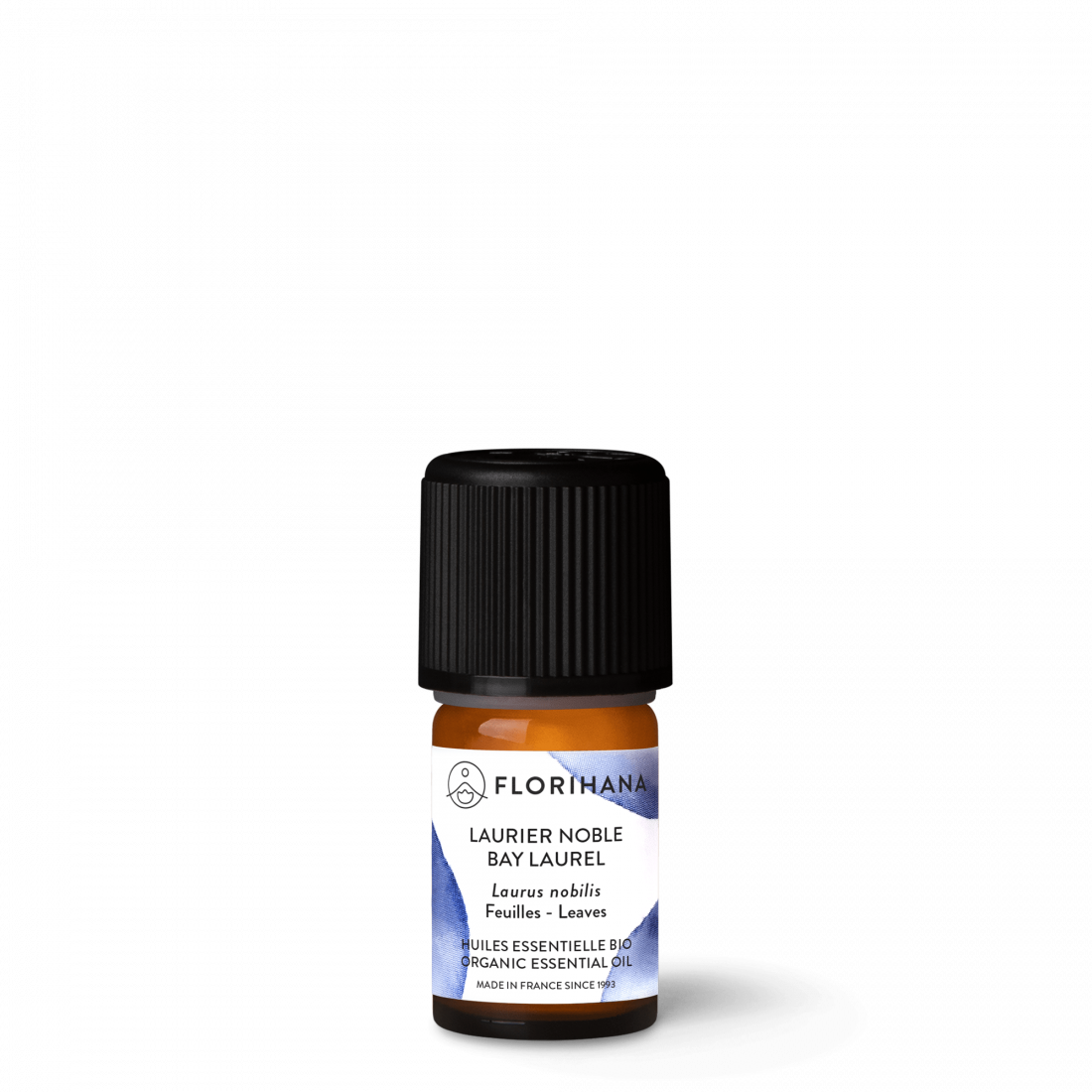This close-up image features a small amber glass bottle of essential oil set against a white background. The bottle, which has a prominent black plastic cap about the same size as the bottle itself, is primarily covered by a detailed label in shades of white and blue. At the top of the label, "Florihana" is prominently displayed alongside a circular logo comprising a pyramid with a circle beneath it. Below, the text reads "L'Oreal Noble Bay Laurel - Laurel Nobilis - Folium Leaves - Bio-Organic Essential Oil," further indicating that the product is made in France since 1993. The oval logo and the distinctive blue circular paint streaks on the label add to the product's distinctive branding.